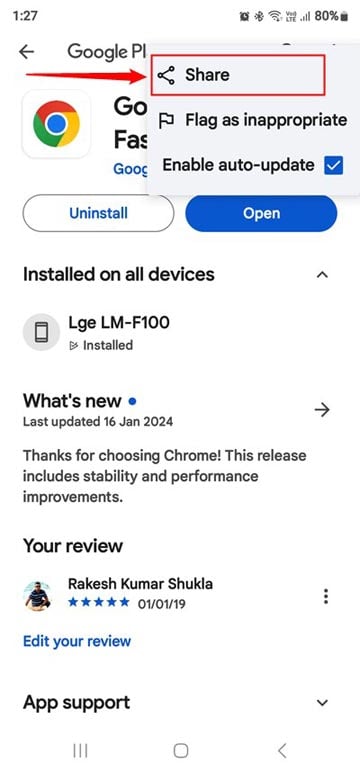This image appears to be a screenshot from the Google Play Store interface. In the upper left-hand corner, there is the number "127" displayed in black text against a white background. The upper right-hand corner showcases several icons: an alarm clock, a full Wi-Fi signal, full mobile data signal, and an 80% battery level.

Directly below, there is a navigation bar starting with a back arrow and the partially obscured text "Google Play" (only "PL" is visible due to a pop-up menu). A red arrow points towards a distinct red outlined block labeled "Share". Beneath the pop-up menu, options such as "Flag as inappropriate" and "Enable auto-update" are visible.

On the left side, the Google Chrome icon is displayed. The interface contains two prominent buttons: a white oval "Uninstall" button with blue text, and a blue oval "Open" button with white text. The description "Installed on all devices" is followed by an upward arrow and the text "LGE LM F100 installed".

Further down, it states "What's new?" along with details about the latest update being on January 16, 2024. The update notes thank users for choosing Chrome and mention improvements in stability and performance.

A review by a user named Rakesh Kumar Shukla, rated 5 stars, is also visible along with the review ID "01019", and options to "Edit your review" or access "App support". Navigation options are partially visible at the bottom which likely include "Back" and "Home screen" buttons.